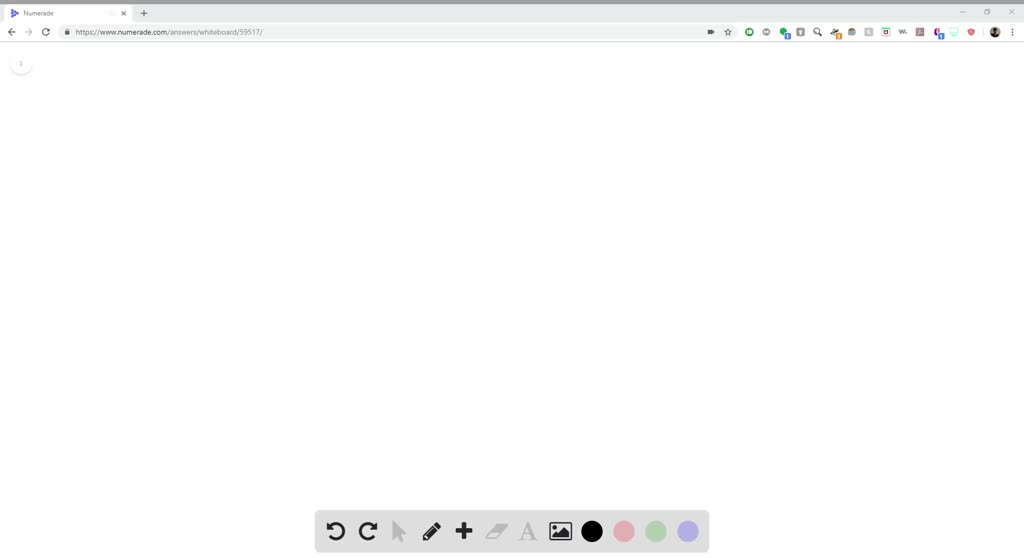This image captures a web browser window showcasing an online painting tool interface. The browser window features a gray bar at the top, housing the back arrow, forward arrow, refresh icon, and the address bar with the website's URL. To the right, typical window control buttons (minimize, maximize, and close) are visible.

Directly beneath the gray bar, the interface displays an array of vibrant icons, shapes, and symbols in red, blue, yellow, and green. These icons are arranged in a toolbar against a white background. Centrally positioned on this white background, there's a prominent grayish bar containing various functional buttons: an undo button, a reapply button, an arrow, a pencil, a plus symbol, an eraser, and a font icon. Additionally, there are color swatches for black, pink, green, and purple, providing users with quick access to these colors for their painting needs.